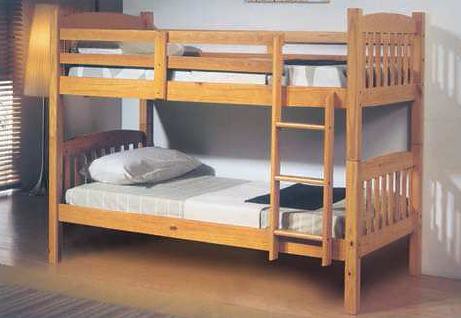The image captures a cozy indoor bedroom setting featuring a sturdy bunk bed with a golden oak wooden frame. The bunk bed, pushed up against a white wall, has a three-step ladder connecting its two tiers. Each tier supports a twin-sized mattress adorned with gray and blue square patterned covers, accompanied by a white puffy pillow. The beds have matching plank headboards and footboards, each detailed with a spindle design and brown wooden railings on the top bunk for safety.

A white cloth drapes from the center of the mattresses, beneath which lies a black pad. The room boasts natural wood floors and features a brown and beige striped throw rug positioned in front of the bunk bed. To the left of the bed is a window, complete with wooden blinds extending down to the floor, allowing natural light to subtly brighten the scene. Adding a touch of warmth, a silver floor lamp with a beige shade stands in the background, casting gentle light over the room and creating soft shadows on the wall. In the corner, a hint of a picture frame is visible above the upper bunk.